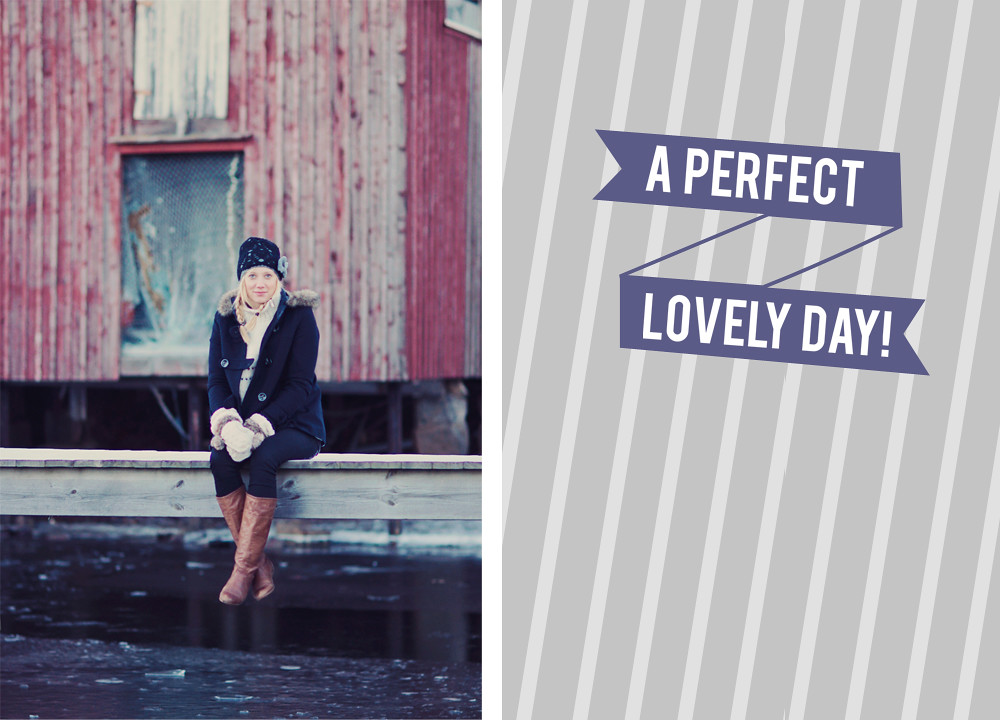The image appears to be a composition of two separate visuals, possibly designed as a card. On the left side, there is a striking photograph of a young woman with blonde hair, dressed warmly in a navy blue peacoat, gloves, mid-calf brown boots, jeans, and a winter cap. She is seated on a white painted wooden bench above what appears to be icy water, indicated by visible patches of ice. The scene suggests a chilly, wintry day. Behind her stands a weathered red barn with a door covered by a net, elevated above the ground, contributing to the rustic charm of the background. The barn's red paint is faded in places, revealing hints of wood beneath and muted tints of red, adding character to the setting. The woman gazes at the camera with a subtle, closed-mouth smile.

On the right side, there is a graphic element characterized by gray and white diagonal vertical stripes. A blue banner bisects the stripes, with the phrase "a perfect" in white text on the top portion. Below, another blue banner reads "lovely day!" also in white text. The design contributes a celebratory and positive sentiment to the overall visual composition of the card.